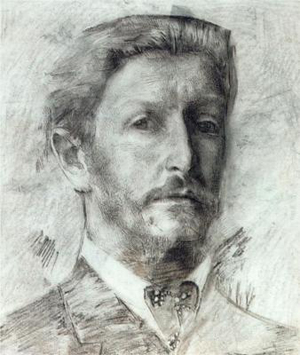This detailed artwork is a distressed charcoal drawing capturing a forward-facing portrait of a serious, middle-aged man. His hair is styled into a slightly slicked-back pompadour, complementing his prominent nose and relatively large ears. A defining feature is his untrimmed, somewhat wild mustache, and possibly a hint of stubble or a beard enhancing his pensive expression. Dressed in a white collared shirt, tie, and jacket, his attire suggests a formal presentation. The background is a gray, smudged expanse, skillfully shaded with the side of the charcoal to create depth and contrast around his shoulders and beneath his chin. Flecks of brown may suggest an intricate mix of pastel or colored pencil details. The overall composition evokes a sense of introspection and solemnity, anchoring the viewer's attention to the man's deep, contemplative gaze.